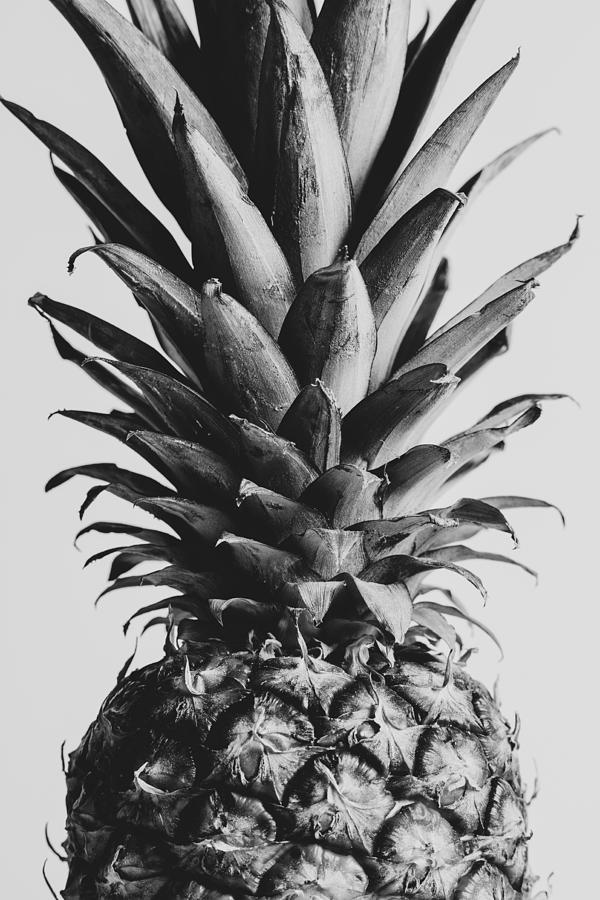This black-and-white portrait-oriented photograph showcases a pineapple, focusing on its upper portion. The composition captures the pineapple from its leafy crown down to approximately halfway through the fruit. The prominent, long, straight, and rigid leaves at the top splay outward, occupying roughly two-thirds of the image's height. Closer to the fruit, the leaves become smaller and slightly curled downward. The fruit itself reveals a segmented surface with thorny, semi-circle patterns and dried wispy ends. The rough, spiked texture of the pineapple's skin is evident. The background is a light gray, with the lighting coming from the right, casting shadows on the left side of the image. The photograph employs a realistic, representational style typical of food photography, emphasizing the detail and textures of the pineapple.